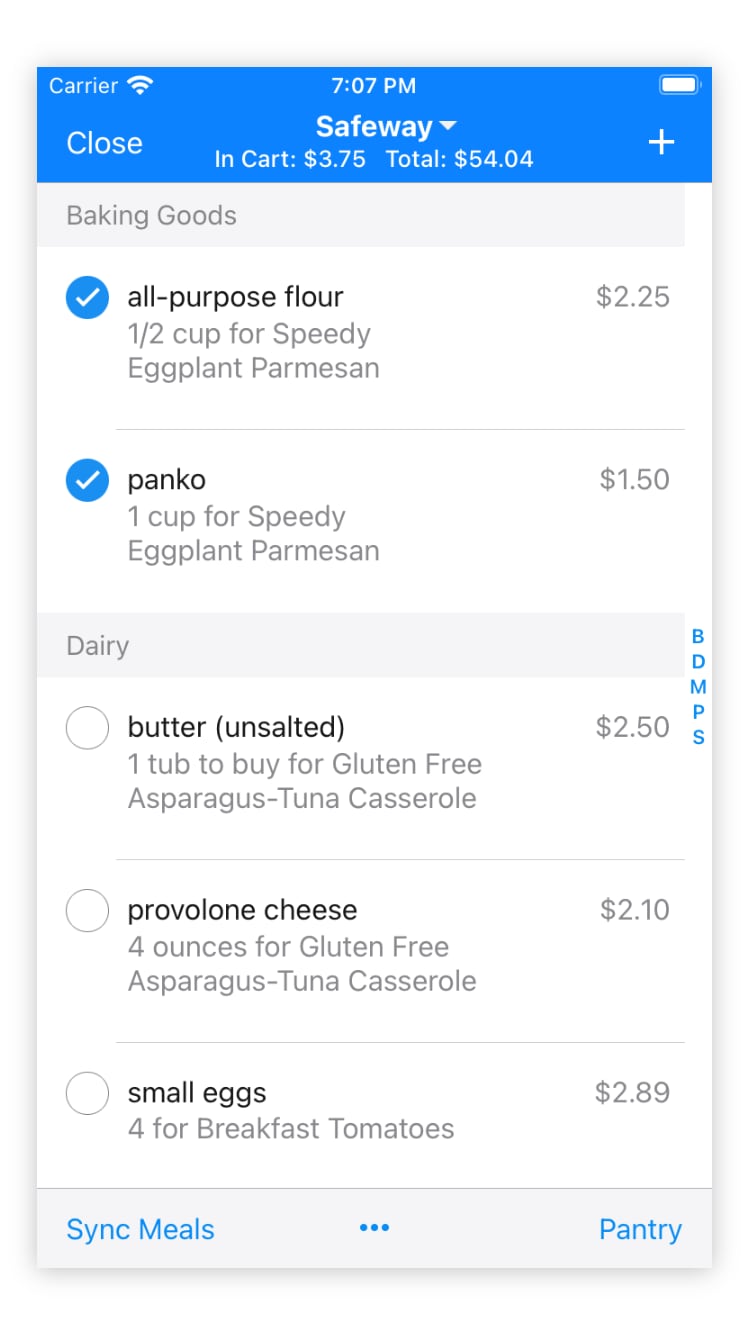This screen capture depicts a grocery order page from a cell phone, displaying the layout and details of a user's shopping cart on the Safeway app. At the very top, within a blue header, the screen indicates the 'Carrier' status along with a Wi-Fi symbol, the time "7:07 PM," and a battery icon on the far right.

Directly below the blue header, the middle part of the screen prominently features the Safeway logo, while the left side says "Close." Under the Safeway logo, the cart summary shows "In-Cart $3.75" and "Total $54.04," with a plus sign icon on the right to possibly add more items.

The first section, labeled "Baking Goods" inside a light gray rectangle, presents items like:
- All-Purpose Flour: Priced at $2.25, marked as "1 1/2 cup for Speedy Eggplant Parmesan," with a blue checkmark circle indicating its selection.
- Panko: Priced at $1.50, marked as "1 cup for Speedy Eggplant Parmesan," also with a blue checkmark circle indicating its inclusion.

Following this, the "Dairy" section lists:
- Butter, Unsalted: Priced at $2.50 for "one tub to buy for Gluten-Free Asparagus Tuna Casserole," without a checkmark, indicating it is not selected.
- Provolone Cheese: Priced at $2.10 for "four ounces for Gluten-Free Asparagus Tuna Casserole," without a checkmark.
- Small Eggs: Priced at $2.89 for "four for Breakfast Tomatoes," without a checkmark.

At the very bottom, there is a light gray footer with multiple navigation options: "Sync Meals" in blue on the left, three dots in the middle, and "Pantry" in blue on the right.